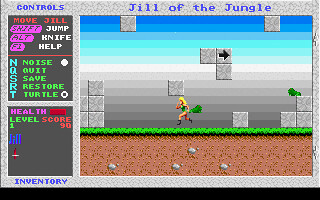This is a detailed screenshot from the classic NES-style video game, "Jill of the Jungle." The game's pixel art showcases a side-scrolling scene where the central character, Jill, is running across a stripe of green grass at the center. Below the grass, the earth is detailed with brown dirt and scattered white rocks, adding to the retro visual appeal. Jill appears to be carrying some leaves, and there are white square stones positioned for her to jump on. 

To the left of the gameplay area, there is a black panel featuring various game stats and controls. This includes instructions such as "Move Jill," "Shift to Jump," "Alt for Knife," and more, including health and level indicators. Above this panel, the word "Inventory" is displayed in blue.

The entire screenshot is bordered by a grey frame. At the top of the frame, on a white banner, the game's title "Jill of the Jungle" is prominently displayed in blue letters. The grey background has a textured, rocky appearance with various shades of grey, adding depth to the scene. The overall layout suggests the game's mechanics and controls, providing an immersive retro gaming experience.